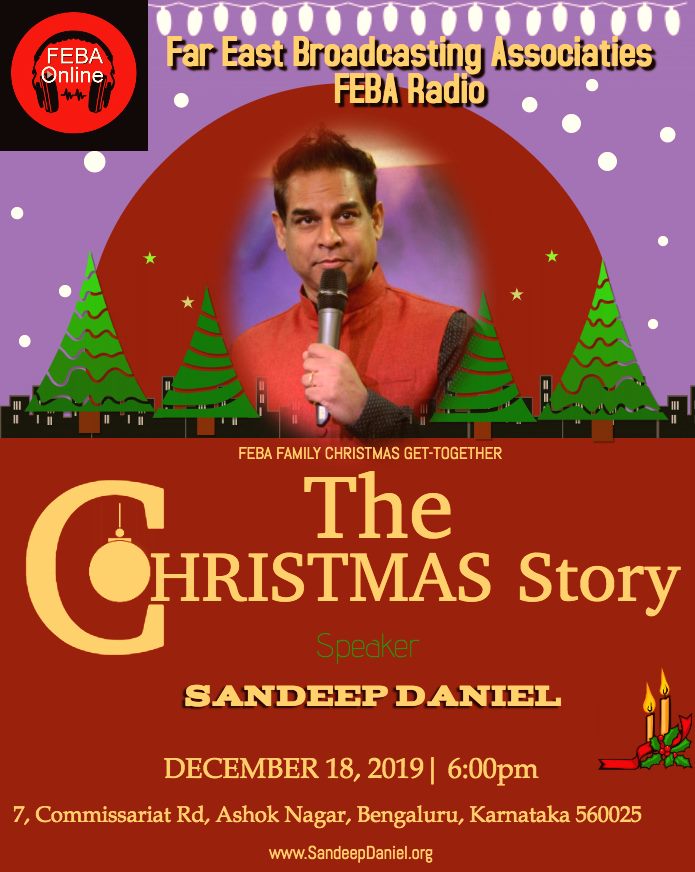The flyer is in a portrait layout, advertising a festive event organized by the Far East Broadcasting Associates (FIBA). The top half of the flyer features a purple background adorned with white lights and tiny dots representing snow. At the very top, a string of Christmas lights adds a festive touch. In the top left-hand corner, the FIBA Online logo, a red circle on a black square with white text and black headphones, is prominently displayed. Central to the flyer is an image of an Indian man wearing a red vest over a gray shirt, holding a microphone, encased in a snow globe-like structure with green Christmas trees flanking him on both sides.

The bottom half of the flyer transitions into a vivid red background with bold yellow text. It details the event: "FIBA Family Christmas Get-Together," followed by "The Christmas Story," with the speaker, "Sandeep Daniel," listed beneath. The event is scheduled for December 18, 2019, at 6 PM, taking place at 7 Commissariat Road, Ashok Nagar, Bengaluru, Karnataka, 560025. Adjacent to Sandeep's name on the left, festive imagery of candles and holly adds Christmas cheer. The flyer also includes the website www.sandeepdaniel.org at the very bottom.